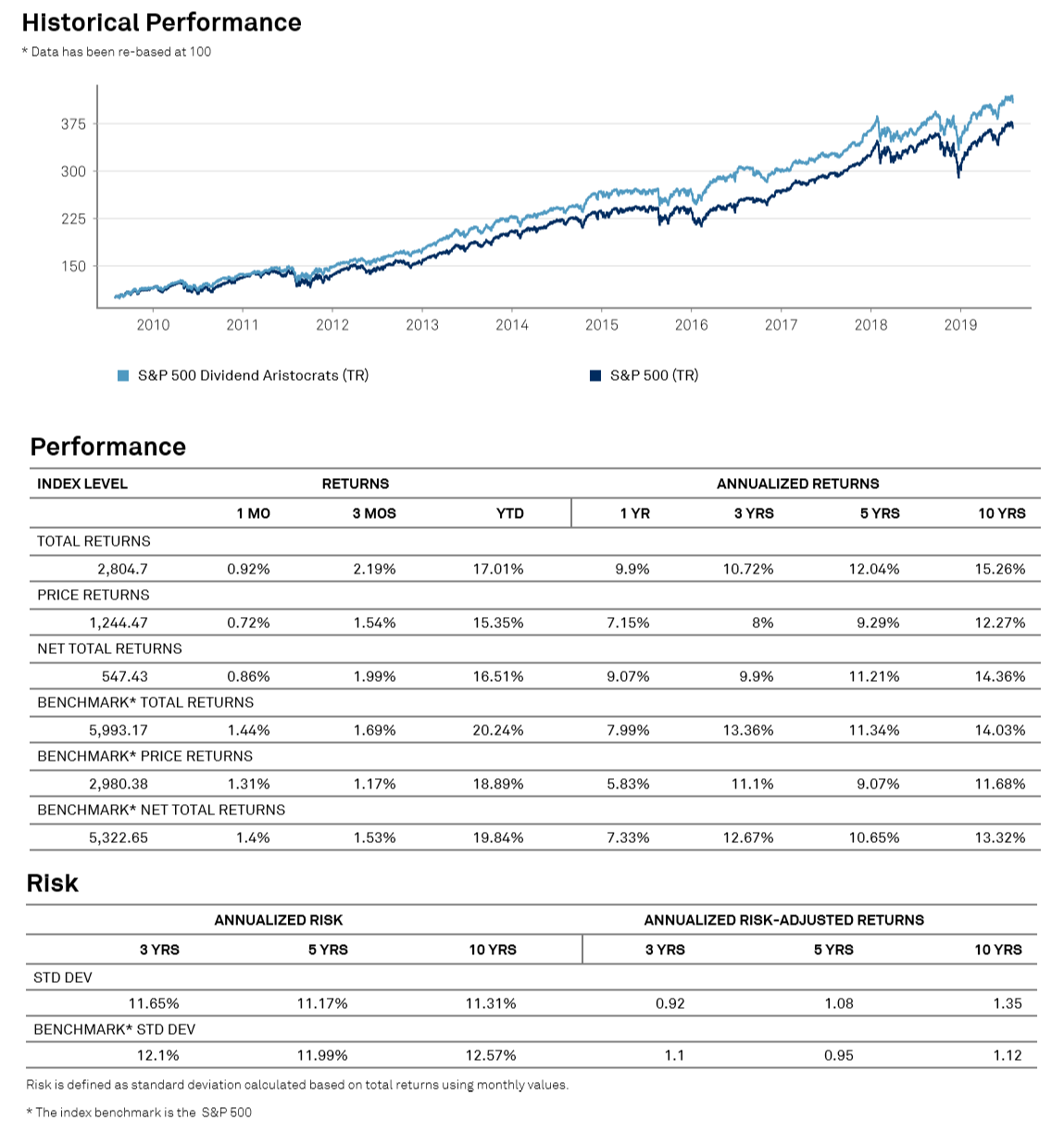**Historical Performance of S&P Dividend Heuristic Rates vs. S&P 500 TR**

The image showcases a comprehensive graph illustrating historical performance data. At the top of the graph, prominently bolded in black with a star next to it, is the label "Historical Performance." All data has been rebased to a value of 100 for comparison purposes.

The vertical axis of the graph is scaled with values 150, 225, 300, and 375, representing performance metrics. The horizontal axis lists years 210 through 219.

The graph exhibits two key performance lines:
1. **S&P Dividend Heuristic Rates**
2. **S&P 500 TR**

These lines trend closely alongside each other, allowing for an insightful comparison of their performance over the designated years.

Beneath the graph, detailed performance levels are provided in an information center, covering various return metrics:
- **Index Returns**
  - Annualized Returns
  - Total Returns: [Insert corresponding data]
  - Price Returns: [Insert corresponding data]
  - Net Total Returns: [Insert corresponding data]
  - Benchmark Total Returns: [Insert corresponding data]
  - Benchmark Price Returns: [Insert corresponding data]
  - Benchmark Net Total Returns: [Insert corresponding data]

The information center also dives into risk assessments, presenting:
- **Annualized Risk**
- **Annualized Risk Adjusted Returns**
  - 3-Year Performance: [Insert corresponding data]
  - 5-Year Performance: [Insert corresponding data]
  - 10-Year Performance: [Insert corresponding data]

Each category is meticulously detailed with corresponding data, providing a thorough analysis of performance and risk over multiple time spans.